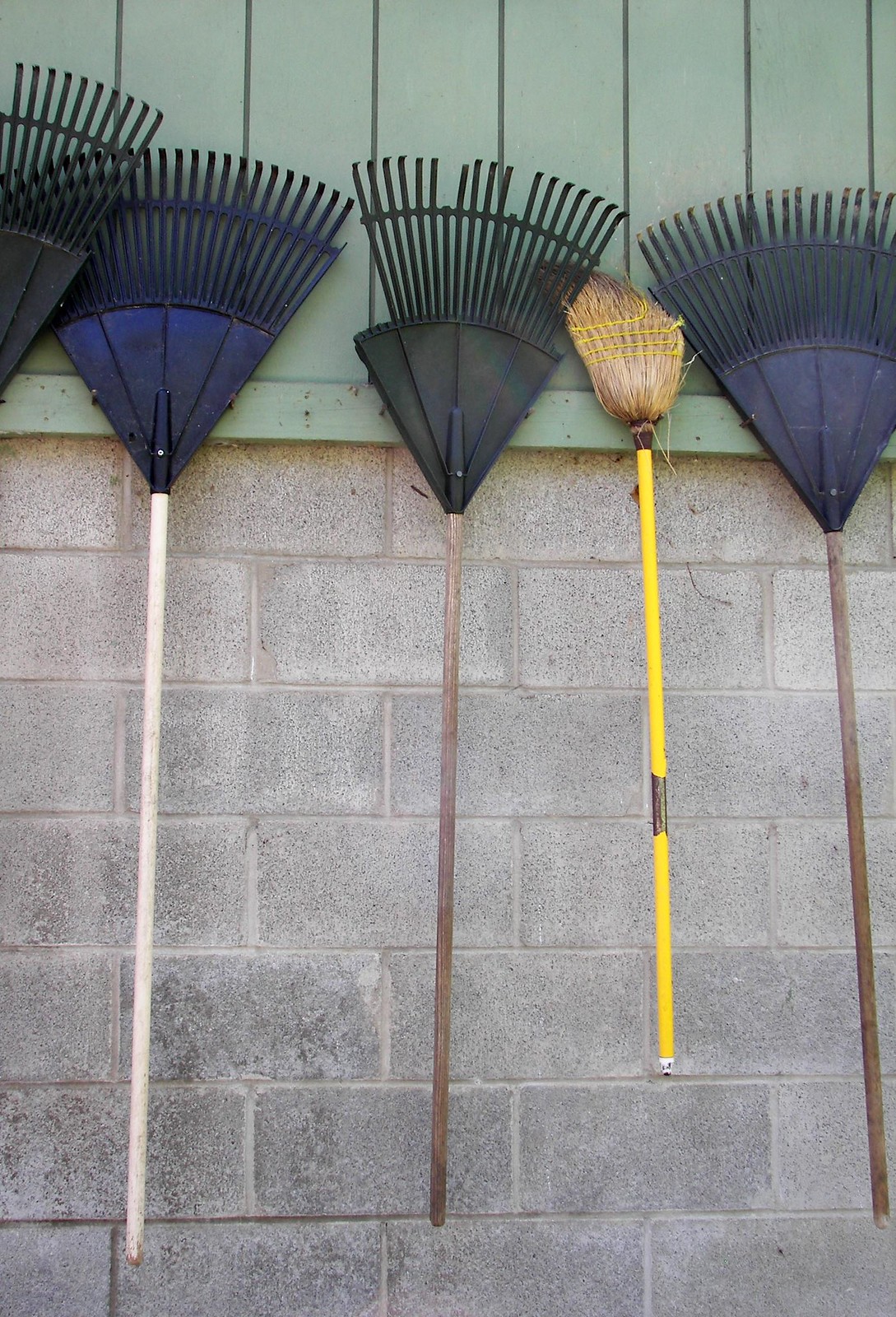This color photograph features a meticulously detailed scene of a shed wall, divided horizontally into two distinct sections: a bottom cinder block base and an upper portion of wide-planked wood painted in a light green hue. The two sections are separated by a 2x4 horizontal beam, which also serves as the mounting board for four nails or hooks.

Suspended from these hooks are four rakes and one broom, each tool showcasing distinct characteristics. Starting from the left, the first visible rake has a white handle and blue tines, partially obscured by the other tools. The second rake also sports blue tines but stands out due to its broken black plastic head, with several tines missing on the left side, and a gray wooden handle. Next is a well-worn corn broom with a vibrant yellow handle, further reinforced with silver duct tape around the grip. The bristles of the broom are noticeably worn at an angle. The final tool on the far right is a wide, blue and black leaf rake with a similarly aged gray wooden handle.

The photograph captures the essence of functional yet weathered tools against the rustic shed backdrop, providing an evocative glimpse into everyday life.